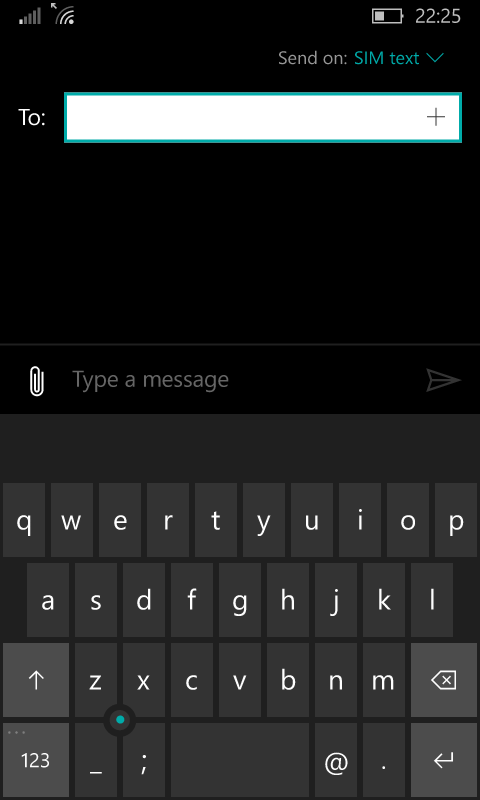The image showcases a mobile screenshot in dark mode, likely due to either user preference or the time of day. In the status bar at the top left, a cellular signal icon with just one bar is visible. Next to it, a Wi-Fi icon with three bars and an arrow pointing diagonally upwards to the left can be seen. The battery indicator shows roughly one-third charge remaining. The time displayed is 22:25, suggesting use of a 24-hour clock format.

Towards the top right, the screen reads “Send on SIM text” in green, indicating that a SIM-based text message is being composed, with a dropdown menu option likely present. Below that, there's a “To” field where a recipient can be entered, and either a plus sign or additional options can be accessed.

Further down on the screen, a paperclip icon signifies the ability to attach files. The phrase “Type a message” is present in the input bar beside a paper airplane icon symbolizing the send button. The keyboard appears in lowercase letters but shows options for uppercase, numeric input, and typical functions like backspace/delete and return. Noticeably, between the “Z” and “X” keys, there is a key combining a hyphen and underscore with a semicolon beneath it. An unusual green circle is also present on the keyboard, though its purpose is unclear. This interface is characteristic of an Android messaging system.